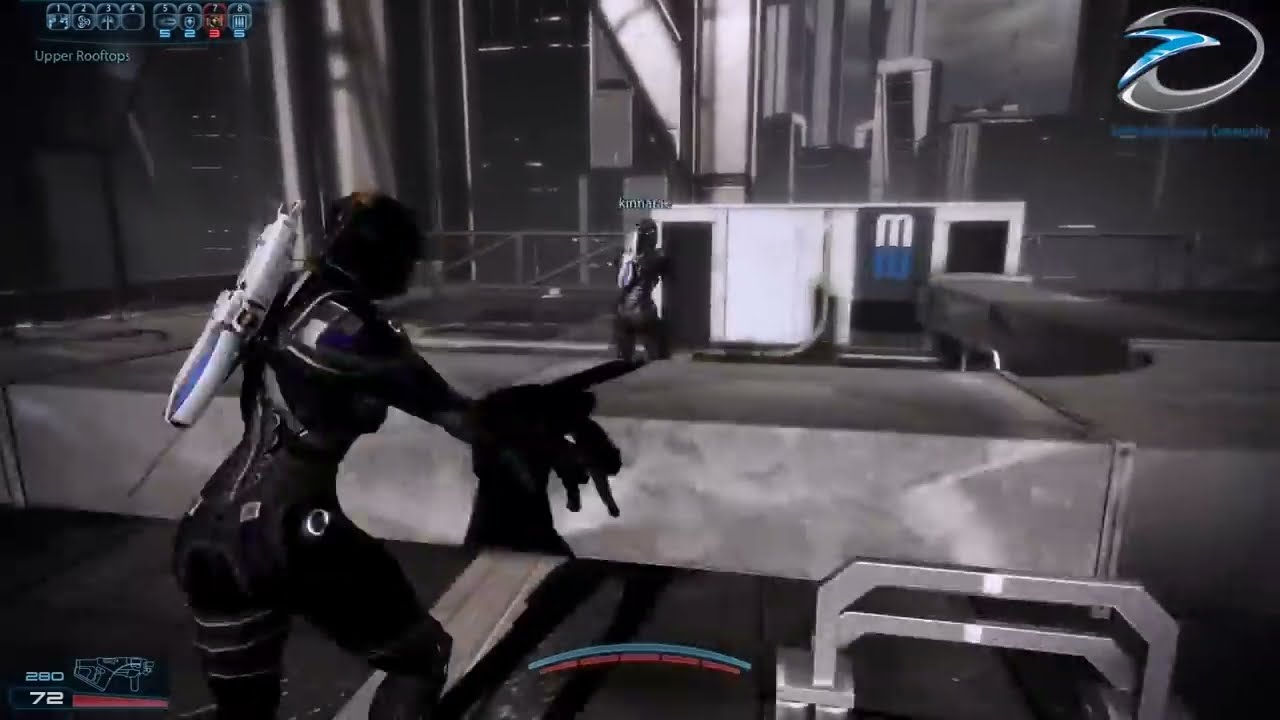The image appears to be a screenshot from a sci-fi video game, captured in a dark, industrial, and futuristic setting. Dominated by shades of gray and black, sporadically broken up by stark shadows and occasional lights, the scene evokes a sense of bleakness and tension. A figure, seen from a third-person perspective, is situated slightly left of center, moving forward. Their features are obscured by shadow, but they carry a rifle on their back, hinting at their potential role as a combatant. 

The screen is cluttered with typical HUD elements: various controls are visible at the top left, while numerical data is shown at the bottom left. More detailed game information, including a health bar at 72%, and an ammo count of 280 rounds, is displayed in the bottom right corner. Additionally, small, barely readable text also appears in the bottom right, including messages such as "nbtn was taken down by geth trooper dogman 75." 

In the background, blurred shapes suggest an ongoing event or explosion, reinforcing the chaotic and dangerous atmosphere of the scene. The overall aesthetic of the game screen is bleakly industrial, with concrete textures and large glass elements adding to the cybernetic ambiance. 

Overall, this detailed HUD and setting hint at a high-stakes, immersive gameplay experience within a gritty, sci-fi world.